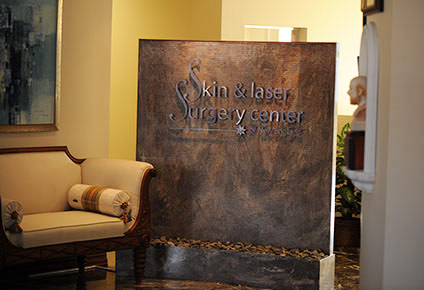The image is taken inside a laser center's waiting room with a retro aesthetic. The room has brown and white walls, and in the background, there's a white fixture resembling an air conditioner. On the left wall, there's a framed abstract painting with shades of blue, above a light gold and dark brown armchair featuring a cream cushion. Central to the image is a large, textured wooden sign with silver lettering reading "Skin and Laser Surgery Center" and a small silver star beneath it. To the right, you can see a bald-headed sculpture with an orange beard, encased in white framing. The room is adorned with dark carpeting and provides a sense of outdated, yet functional, decor typically seen in a doctor's office.